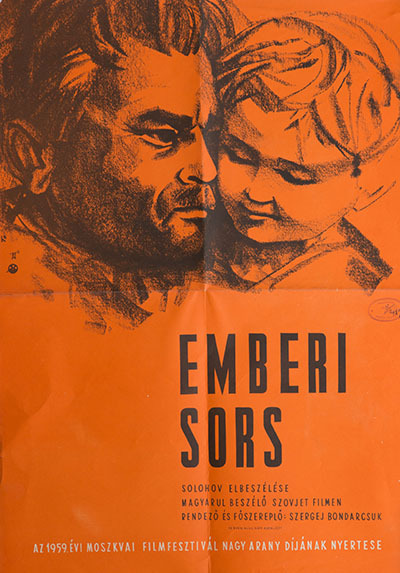This image depicts a poster that features a bright orange background with a detailed charcoal sketch of a man and a young boy’s faces. The man has dark features, including a dark beard, mustache, bushy eyebrows, and messy dark hair; he wears a stern expression and is looking slightly away. The young boy, who has lighter, short hair, appears to be smiling gently and has his eyes slightly closed, snuggled closely against the man's face, suggesting an intimate, possibly familial bond. Beneath the drawing, the title "Emberi Sors" is prominently displayed in bold black letters. Below this title, there are three lines of text in a different language, possibly providing credits or further information about the stars. At the bottom, a row of smaller white text likely includes additional details such as the film festival name or release year. The poster, which seems to be folded into four quadrants, hints at a somber drama, possibly produced around 1959 and related to Moscow.